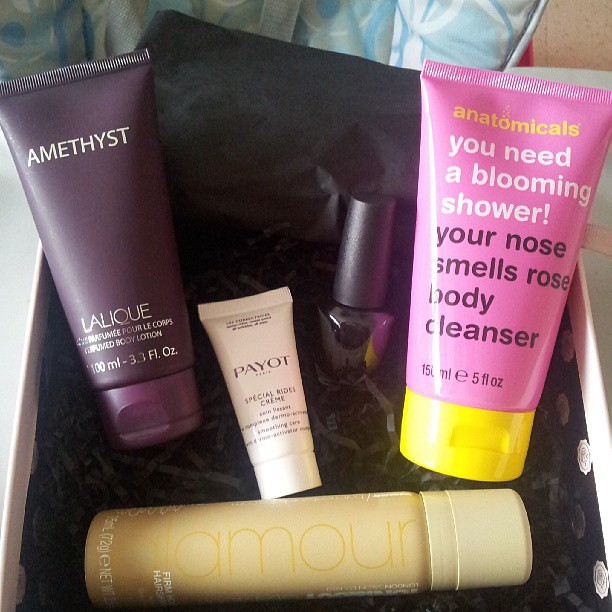This image depicts an open box filled with various cosmetic products, protected by black, confetti-like paper shreds. The white box edges are visible, framing five distinct items. Starting from the left, there is a purple bottle labeled "Amethyst Lalique Body Lotion," which appears to be 3.3 oz (100 ml). Next is a small white container labeled "Payot Special Rides Cream." Following that is a black nail polish bottle. To its right is a large pink tube with a yellow cap, labeled "Anatomicals You Need a Blooming Shower. Your Nose Smells Rose Body Cleanser," with both white and yellow text. The final item, positioned near the bottom, is a beige bottle with the word "Glamour" on it.